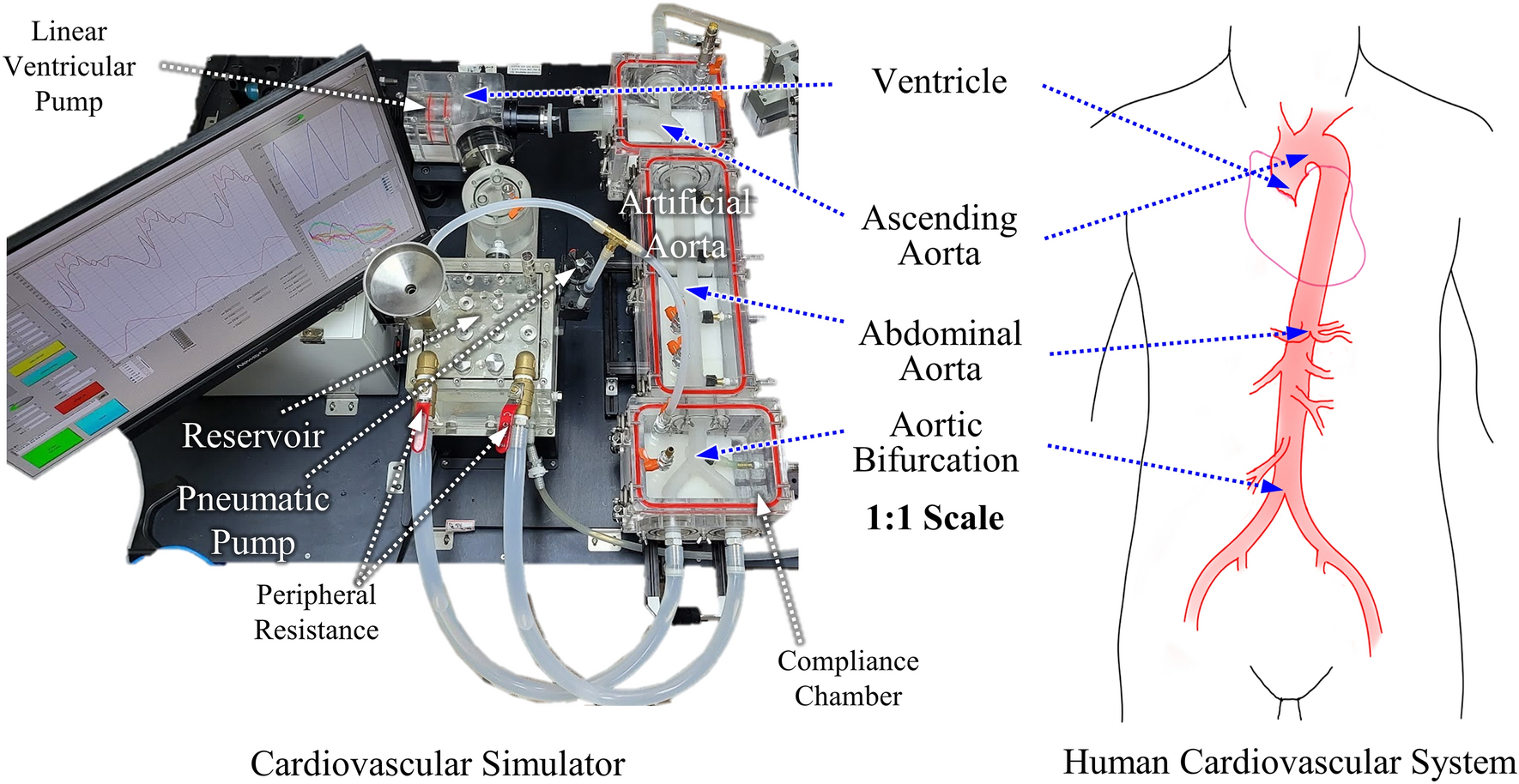This image features a detailed comparative illustration of a cardiovascular simulator and a human cardiovascular system. On the left, the cardiovascular simulator is depicted with lifelike precision, showcasing various mechanical components such as an artificial aorta, linear ventricular pump, reservoir, pneumatic pump, and peripheral resistance. This simulator, designed to mimic the function of the human heart, includes a computer screen that charts relevant data, enhancing its educational utility.

On the right, a simplified line drawing of the human cardiovascular system is presented. This schematic outlines the key elements of the system in red against a white and black background. It highlights significant parts like the ventricle, ascending aorta, abdominal aorta, and aortic bifurcation, all labeled with blue arrows and text. The two depictions are meticulously labeled and connected, allowing for direct comparisons between the simulator’s mechanical components and their biological counterparts. Both representations adhere to a one-to-one scale, emphasizing precise correlations and facilitating a deeper understanding of cardiovascular mechanics.